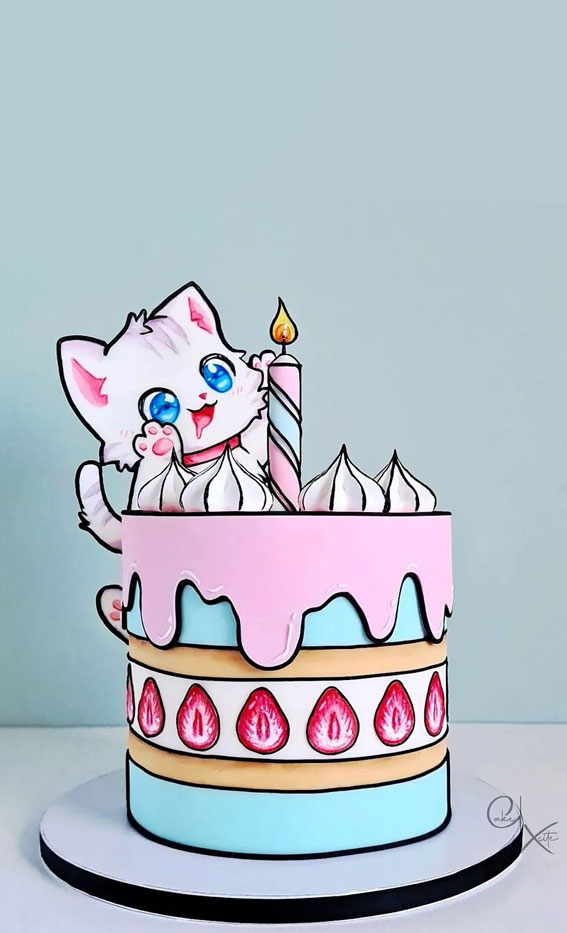In this detailed and vibrant illustration on a light green background transitioning to gray towards the bottom right, a whimsical, three-tiered birthday cake commands attention. The cake rests on a round blue base with a pronounced black stripe, placed on what appears to be a gray countertop. The bottom tier of the cake is teal, followed by a middle white tier adorned with bright red strawberry slices, and topped with another teal layer. Each tier is meticulously trimmed in black, adding contrast and depth. Dripping from the top is a luscious, light pink frosting, decorated with delicate white meringue swirls, also trimmed in blue. A charming blue-and-white striped candle with a yellow flame stands proudly at the cake's peak. To the left, a gleeful white kitty with big blue eyes and a pink tongue lolling out watches the candle. The kitty's ears are pink inside, and it has a small tail sticking out. The ambiance is playful and celebratory, completed by the artist's initials, "CX," in the bottom right corner of the background.